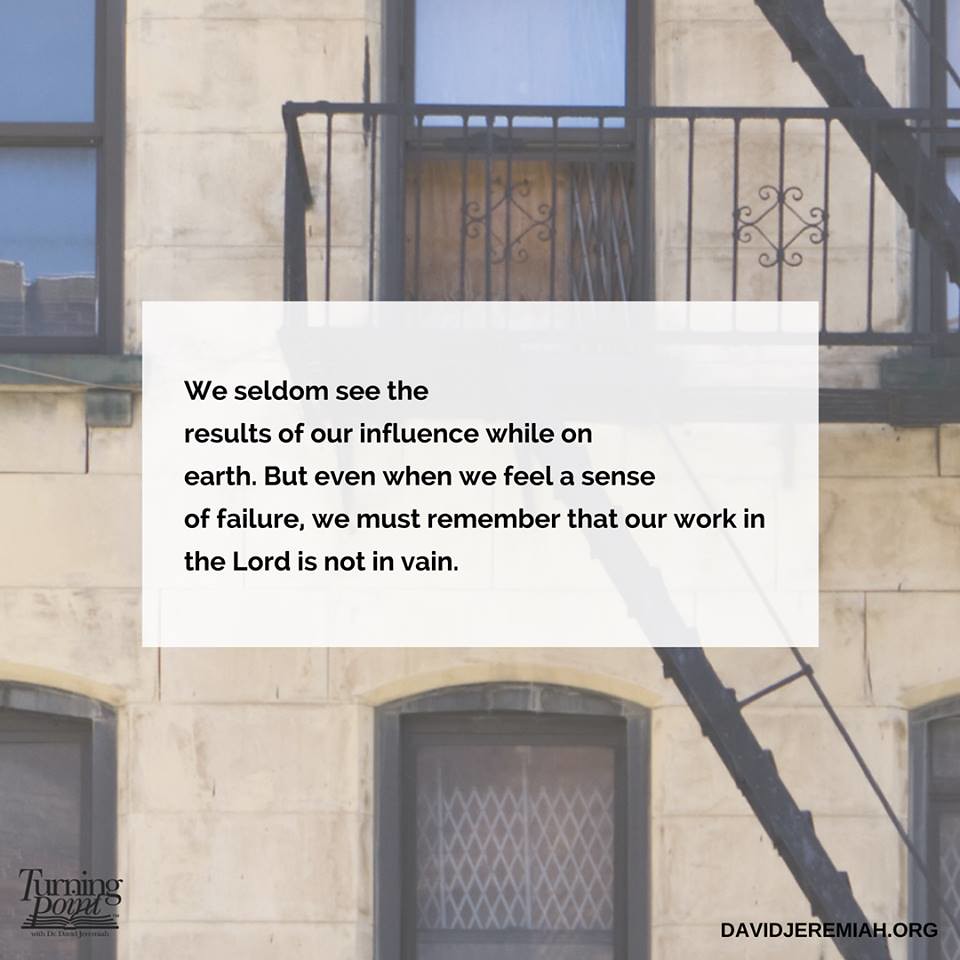The image depicts a brick apartment building with at least two stories, identifiable by two sets of windows, one above the other. A metal staircase extends from a balcony and leads downward. Prominently overlaid in the center of the image is a white rectangle containing a black font quote that reads, "We seldom see the results of our influence while on earth, but even when we feel a sense of failure, we must remember that our work in the Lord is not in vain." In the lower right corner, the black font text "davidjeremiah.org" is visible, along with the term "Turning Point," indicating the source of the quote.